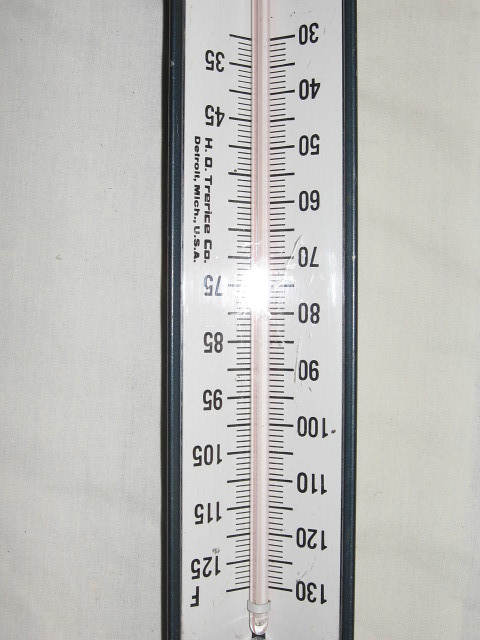This photograph captures a vintage thermometer, charmingly presented upside down. The backdrop features a muted grayish lilac hue, complementing the black-framed thermometer with its subtly V-shaped sides. Encased within this frame is a clean white background, adorned with black lettering.

Despite its inverted position, it is observed that near the top left of the thermometer there are the markings 'H-D-T-R, possibly 'E-R-I-C-E CO.', followed by 'Detroit, M.I.C.H., U.S.A.'—hinting at the device's antiquity through the old-fashioned state abbreviation.

The thermometer has two scales: the left side (viewed in this orientation) measures Fahrenheit, marked with an 'F' at the lower end, and the right side shows a corresponding centigrade range, though without a designated 'C'. The Fahrenheit scale displays measurements at intervals: 35, 45, 75, 85, 95, 105, 115, and 125 degrees. Conversely, the centigrade scale is incremented more uniformly at 30, 40, 50, 60, 70, 80, 90, 100, 110, 120, and 130 degrees.

Central to these markings is a slender glass tube, light pink in color, devoid of any visible indication of the current temperature. This tube would traditionally house mercury or a similar substance for temperature measurement. The overall composition of this image, with its detailed background and vintage thermometer, evokes a nostalgic glimpse into historical meteorological instruments.